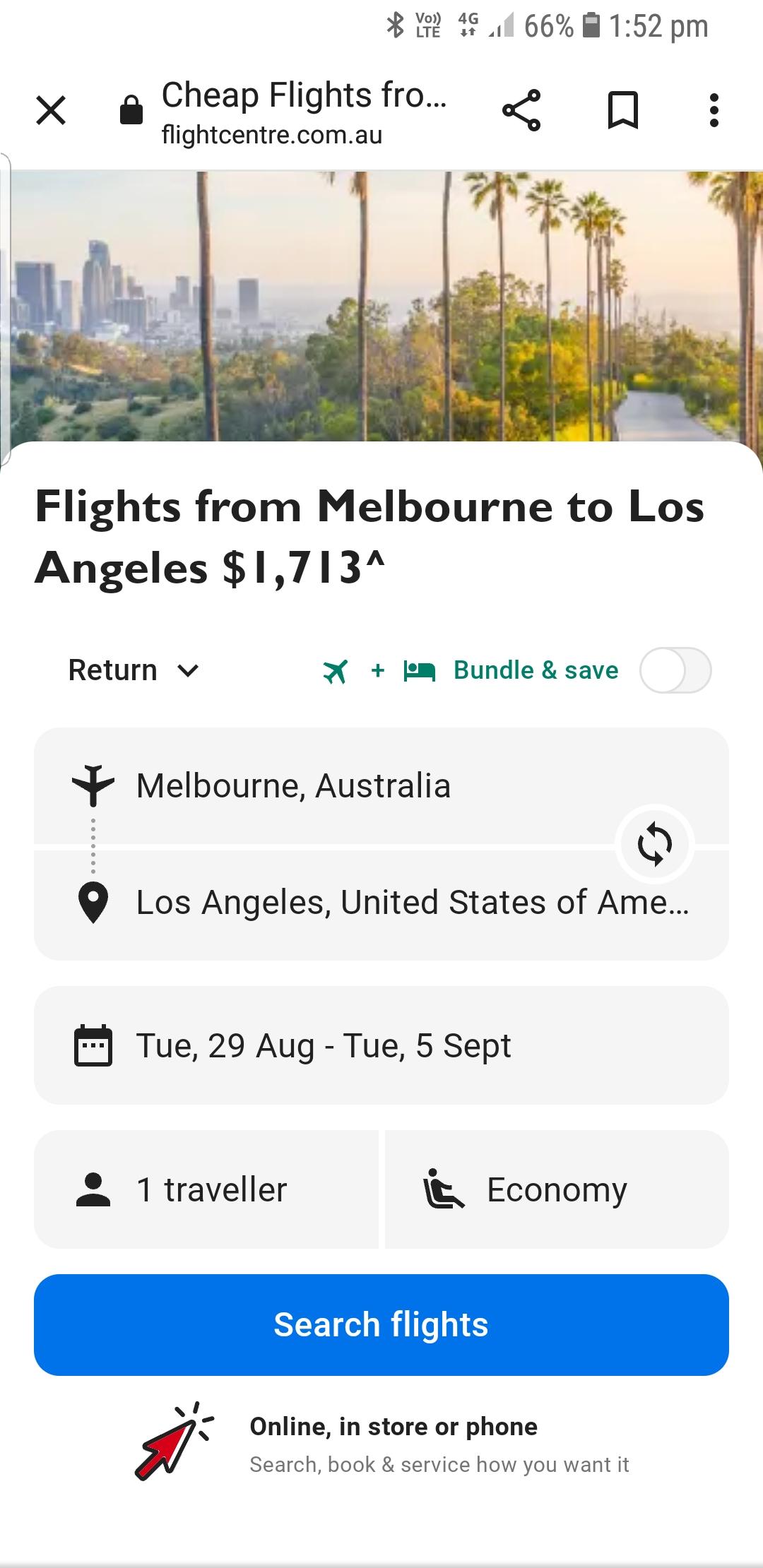A screenshot from a smartphone displays a webpage where someone is searching for flights from Melbourne, Australia to Los Angeles, United States. The one-way flight is scheduled for Tuesday the 29th, with a return flight on Tuesday, September 5th. At the top of the screenshot, the header reads, "Cheap Flights from," though "MN" is partially cropped out. The webpage is from flightcenter.com.au, advertising flights from Melbourne to Los Angeles for $1,713. 

Beneath this, options to select return flights are available, alongside a green plane icon and a "bundle and save" suggestion featuring someone sleeping in a bed. Near the bottom of the page, there's a "Search Flights" button, alongside options to book online, in-store, or by phone, with a tagline reading "Search, book, and service how you want it."

The smartphone's status bar is visible, showing the time, battery life and percentage, Wi-Fi connection, 4G network availability, and Bluetooth status. The interface also allows users to switch the departure and arrival cities between Melbourne and Los Angeles.